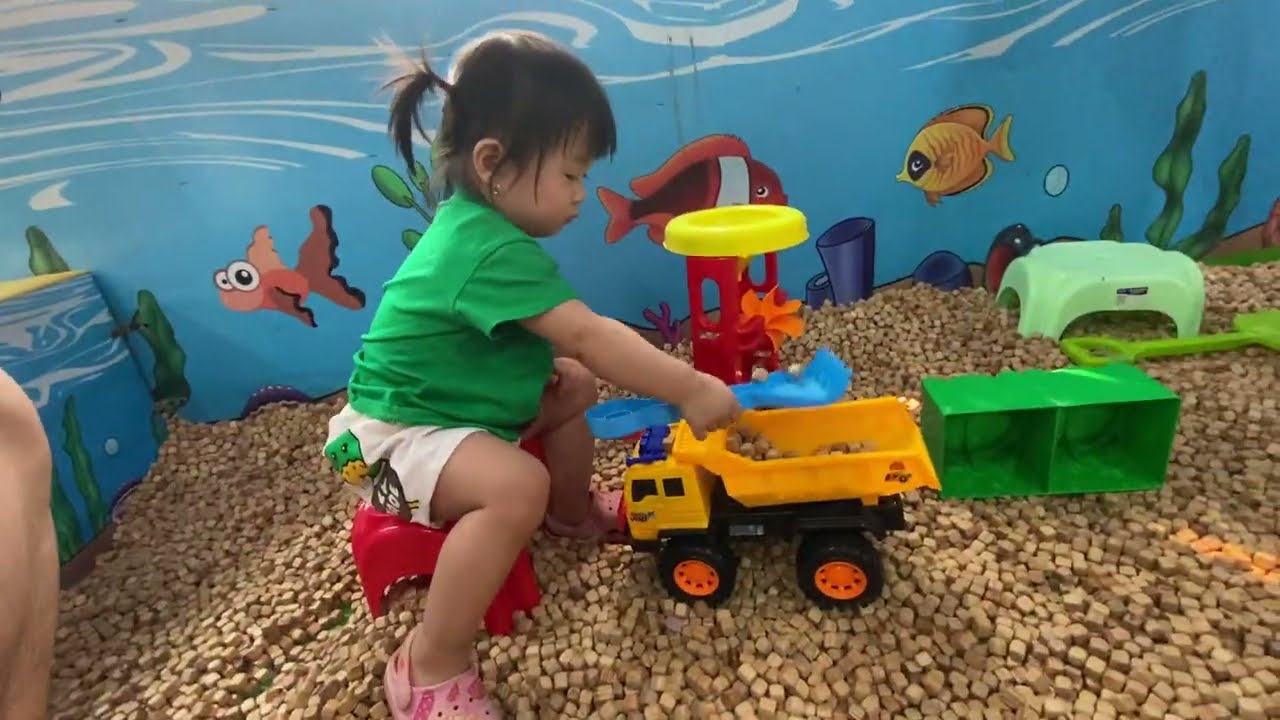A young Asian girl, appearing to be around 3 years old, is playing in an outdoor playground area filled with light tan, cube-shaped wood chips scattered on the ground. She sits on a small red plastic stool, dressed in a green short-sleeved t-shirt and white shorts adorned with a small green duck print. Her dark brown hair is styled in pigtails, and she wears pink Crocs on her feet. In front of her, she shovels wooden blocks into a yellow toy dump truck, surrounded by a variety of colorful toys, including shovels and a green plastic tub. The background features an underwater-themed mural with blue water, tropical fish in yellow and orange, and green algae, enhancing the playful aquatic atmosphere.